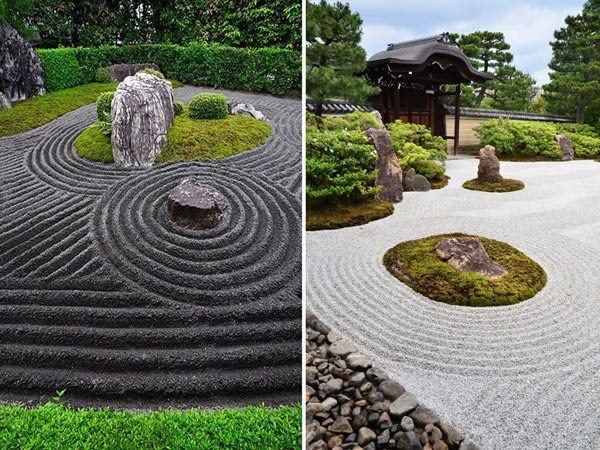This image consists of two side-by-side photographs of intricately designed Zen Gardens. The left-hand photograph showcases a terraced garden with a dark gray or black sand base, meticulously raked into circular patterns. Nestled in this sand is a large rock and a green, circular patch of grass with another rock at its center. The foreground is green, possibly grass or ground cover, and the background features beautifully manicured bushes and trees that form a hedge, stretching across the image.

On the right-hand side of the image, the Zen Garden contrasts with its white sandy landscape, also adorned with raked patterns and circular designs. Central to the design is a flat rock surrounded by grass, with another rock standing prominently amidst the circular grass patches. Further into the image, there is a structure resembling a gazebo or cottage with a Japanese architectural style, made from dark wood. Surrounding the garden are well-trimmed shrubs and trees, completing the serene and meticulously maintained landscape. The overall contrast between the black and white sands, combined with the intricately raked patterns and thoughtfully placed rocks and foliage, creates a harmonious and detailed depiction of the gardens.